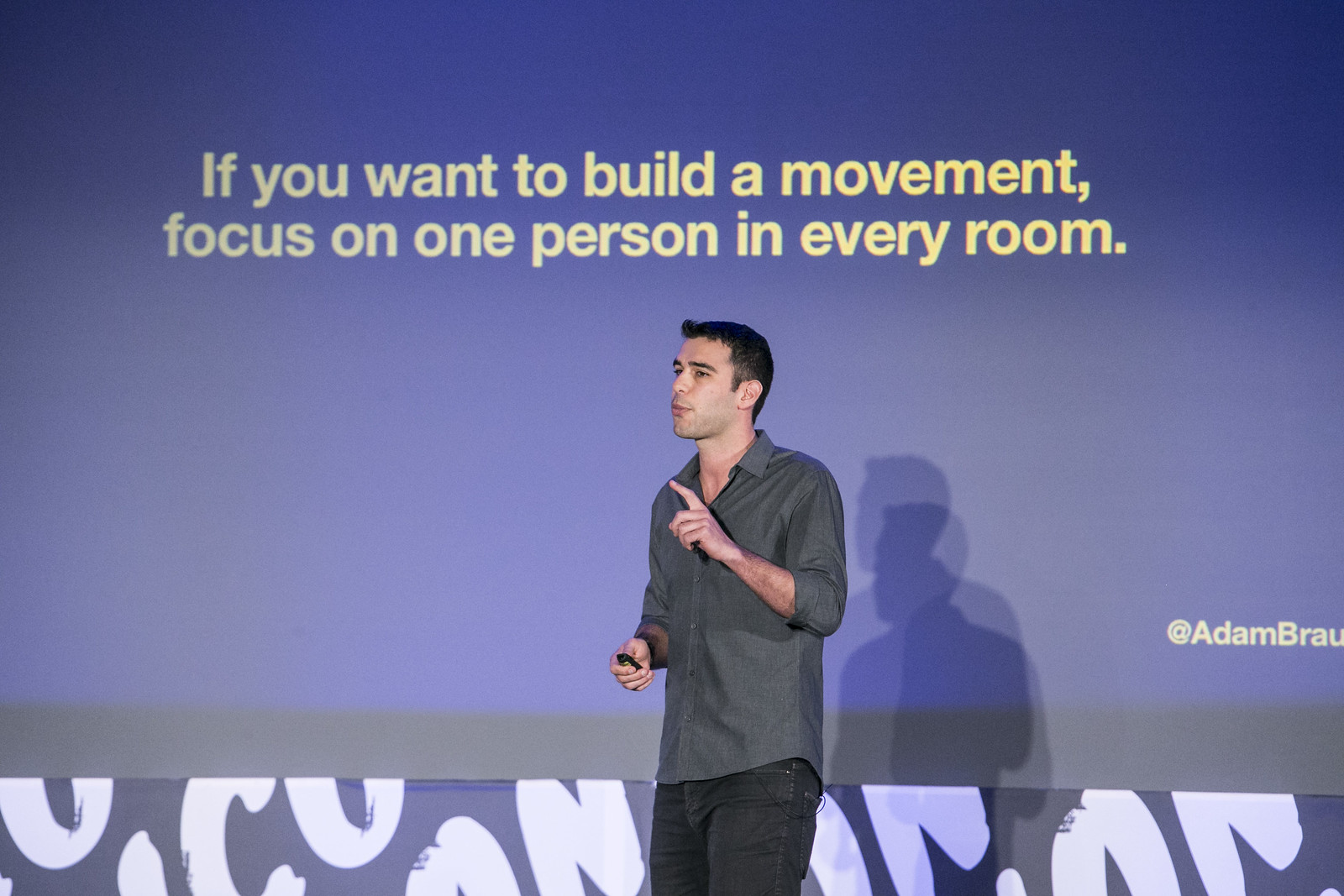A young man with short black hair is seen speaking to an audience at a conference. He is holding a controller in his right hand, seemingly operating a projector that displays text on a large screen. The screen has a blue background with the words, "If you want to build a movement, focus on one person in every room," prominently projected. A shadow of the young man is visible behind him, adding depth to the scene. In the bottom right corner of the screen, part of a logo is visible, reading "At Adam, B-R-A-U," but the complete logo isn't fully shown. The young man is dressed in a long-sleeve green sports shirt and black jeans. He stands confidently in front of the audience, engaging them through his presentation.